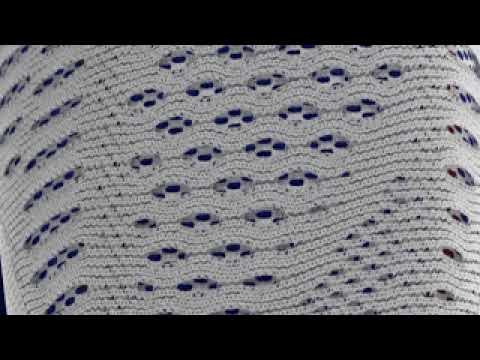The image features a detailed close-up of a white knit fabric with intricate patterns, possibly made from wool and showcasing various levels of transparency. The knit exhibits a repeating diamond pattern where within each diamond, there are four smaller circles. This design creates areas where the fabric is more and less see-through, revealing a blue fabric underneath, adding dimension to the image. The fabric appears to be wrapped around something, possibly suggesting the contour of a back or a vertical column. The borders of the image are black, framing the fabric, which might be part of a shawl, sweater, or possibly a loose blanket. The photograph captures the complexity and meticulous nature of the knit pattern, emphasizing the craftsmanship involved.